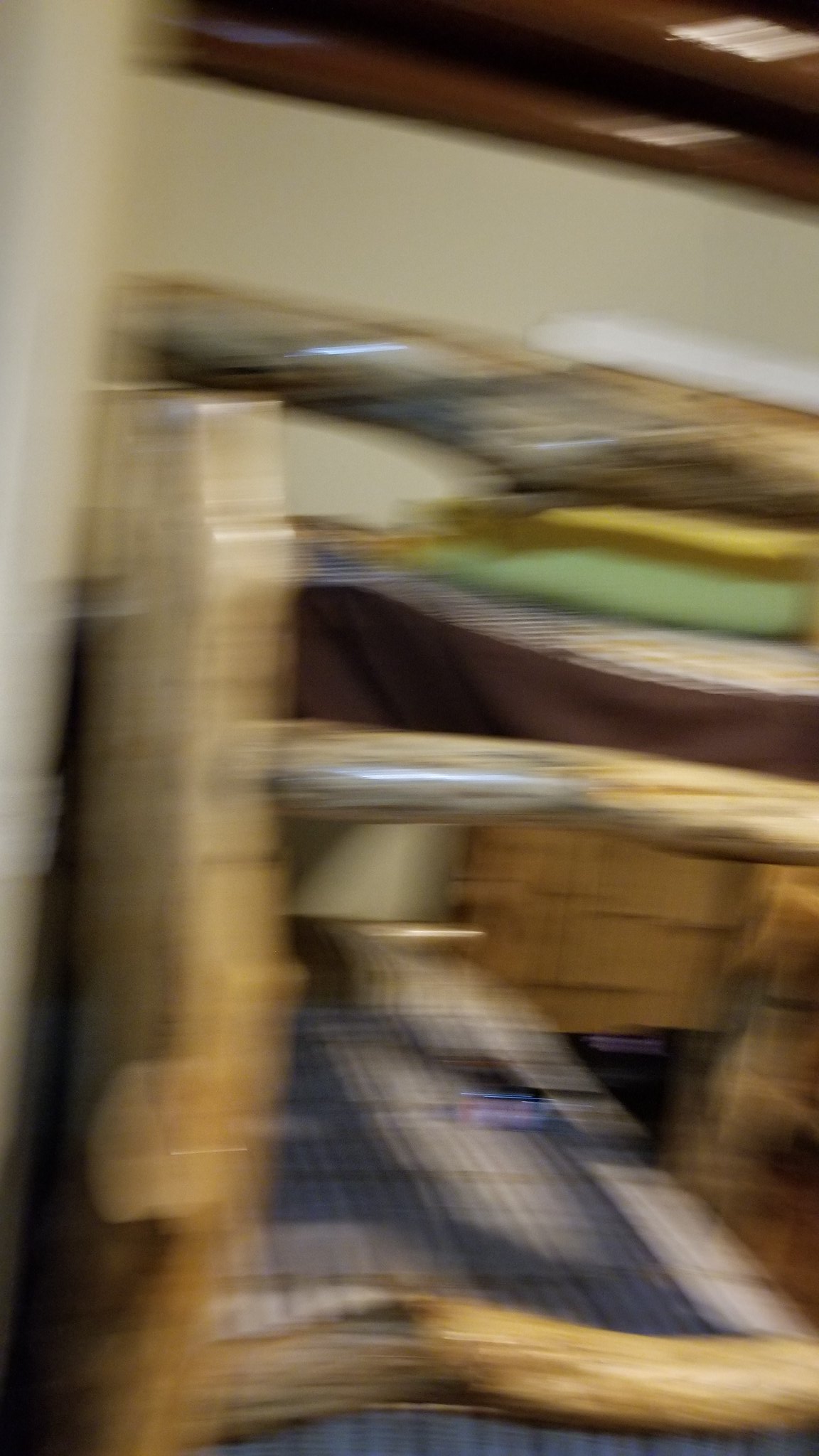This rectangular portrait photograph is notably blurry, creating a sense of mystery and abstraction. Dominating the upper portion, there's a brown section that diagonally stretches from the top left towards the bottom right. Below it lies a defined white rectangular piece, adding a stark contrast to the composition. In the foreground, a light brown wooden object, turned on its side, adds a rustic element. Scattered throughout the image, accents of various colors—blue, white, green, yellow, and light purple—offer a vibrant spectrum, although their shapes and forms remain indistinct due to the blurriness. The overall image presents a vivid yet enigmatic interplay of textures and hues.